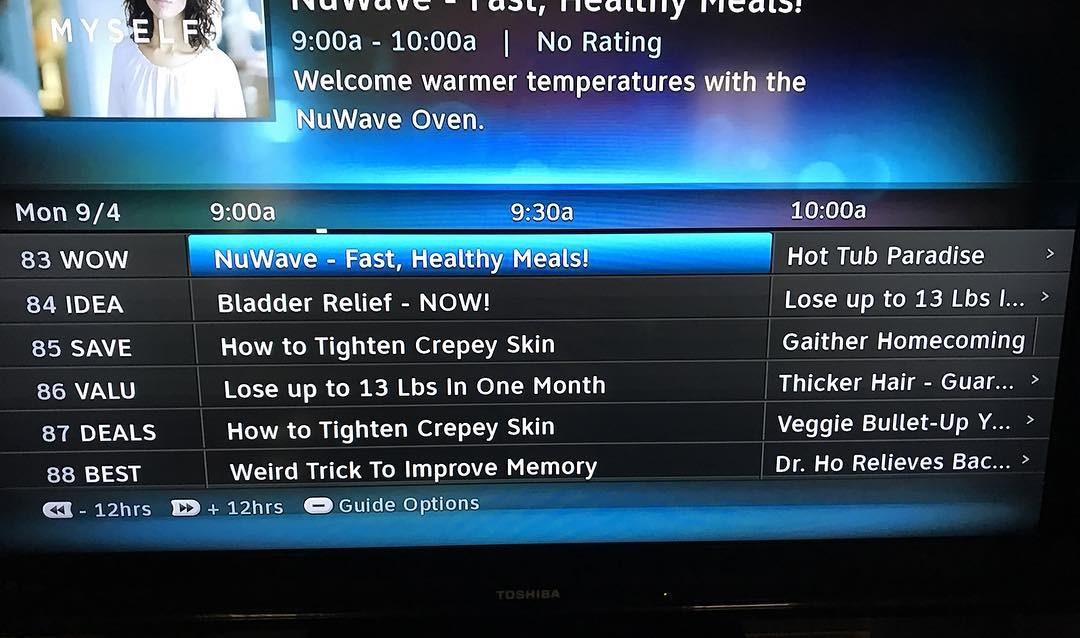This is a highly detailed photograph of someone's TV screen displaying a cable guide for Monday, September 4th, from 9:00 AM to 10:00 AM. The image features a typical TV guide interface, with a blue background at the top displaying a segment's details and a visual on the left showing a woman with curly brown hair wearing a white peasant-style shirt. Superimposed on the visual is a heading that reads "New Wave Fast Healthy Meals" scheduled from 9:00 AM to 10:00 AM, with a note below indicating "no rating" and a promotional message: "Welcome warmer temperatures with the New Wave Oven."

Beneath this promotional area, the guide lists various channels and their respective programs. The channel numbers and programs are in three columns under the date header "MON 9/4" with the time slots clearly marked. At 9:00 AM, channel 83 (WOW) is showing "New Wave Fast Healthy Meals," channel 84 (Idea) has "Bladder Relief - Now!", channel 85 (Save) features "How to Tighten Crepey Skin," channel 86 (Value) airs "Lose Up to 13 Pounds in One Month," channel 87 (Deals) repeats "How to Tighten Crepey Skin," and channel 88 (Best) shows "Weird Trick to Improve Memory."

For the 10:00 AM slot, channel 83 will air "Hot Tub Paradise," and subsequent channels follow with different shows: channel 84 continues with "Lose Up to 13 Pounds," channel 85 with "Gather Homecoming," channel 86 with "Thicker Hair," channel 87 will show "Veggie Bullet," and channel 88 listing "Dr. Ho Relieves Back Pain." 

At the bottom of the screen, there is a black border with "Toshiba" written in white letters, indicating the brand of the TV.